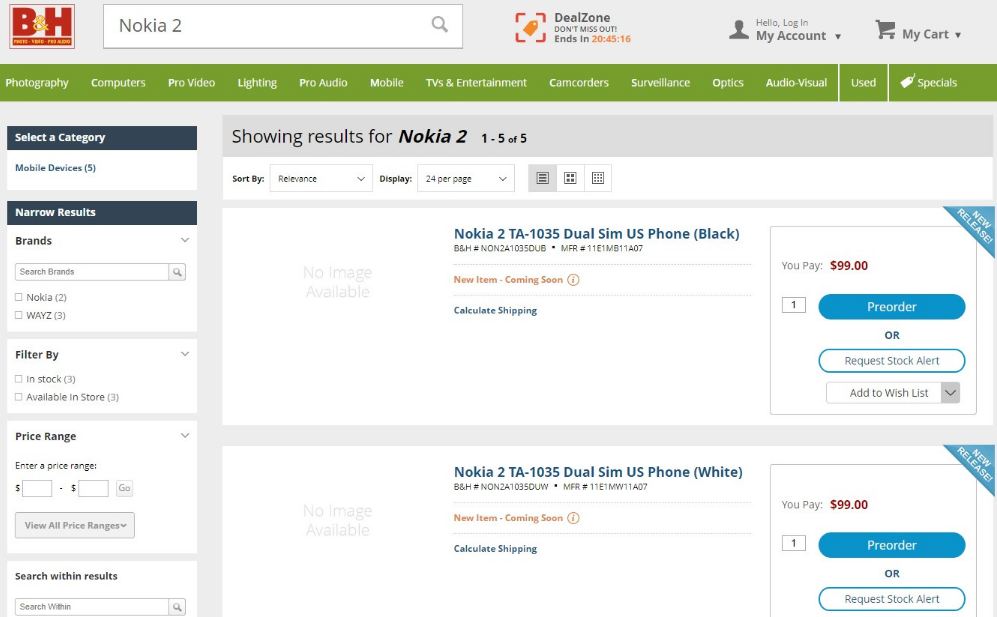The image displays the website header and interface of the BNH store. At the top, there is a grey header with the text "BNH" on the left. On the right side of the header, there is a search bar containing the text "Nokia 2." Next to the search bar, there is a "Deal Zone" section accompanied by a countdown timer. The top right corner features text options "Hello, Login" and "My Account" alongside a dropdown menu and a shopping cart icon labeled "My Cart."

Beneath the grey header, there is a green navigation menu with categories listed from left to right, including: "Photography," "Computers," "Pro Video," "Lighting & Pro Audio," "Mobile," "TV & Entertainment," "Camcorders," "Surveillance," "Optics," "Audio-Visual," "Used," and "Specials."

Below the navigation menu, search results for "Nokia 2" are displayed, showing 1 of 5 results. The first result indicates "No Image Available" and describes the product as "Nokia 2 TA-1035 Dual SIM US Phone (Black)." The product details include a price of $99 and a blue "Pre-Order" button.